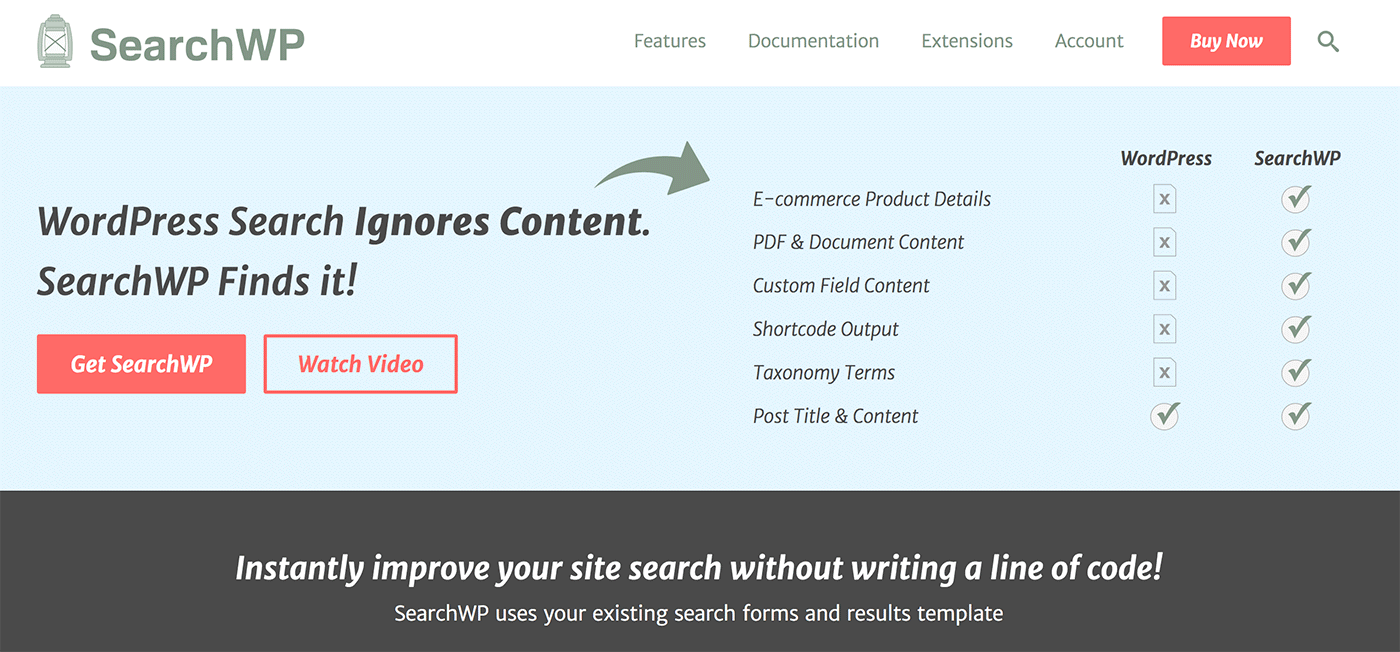In the upper left-hand corner of the image, there's a logo featuring the letter "X." Adjacent to the logo, "Search WP" is written, with 'Search' in capitalized green letters and 'WP' fully capitalized. Moving rightward, there are smaller links labeled "Features," "Documentation," "Extensions," and "Account," followed by a prominently shaded rectangular "Buy Now" button. Immediately to the right of this button is a magnifying glass icon.

The page's main content starts on the left side, where the phrase "WordPress Search ignores content" appears, with "ignores content" in bold. Directly below, it reads "Search WP finds it." Beneath these statements, there are two clear rectangular buttons labeled "Get Search WP" and "Watch Video."

At the bottom of the webpage, a message reads: "Instantly improve your site search without writing a line of code. Search WP uses your existing search forms and results template." On the right-hand side, there is a feature comparison chart between WordPress and Search WP. The chart shows that Search WP includes features like e-commerce product details, PDF and document content, custom field content, shortcode output, taxonomy terms, and post title and content, whereas WordPress only checks off post title and content.